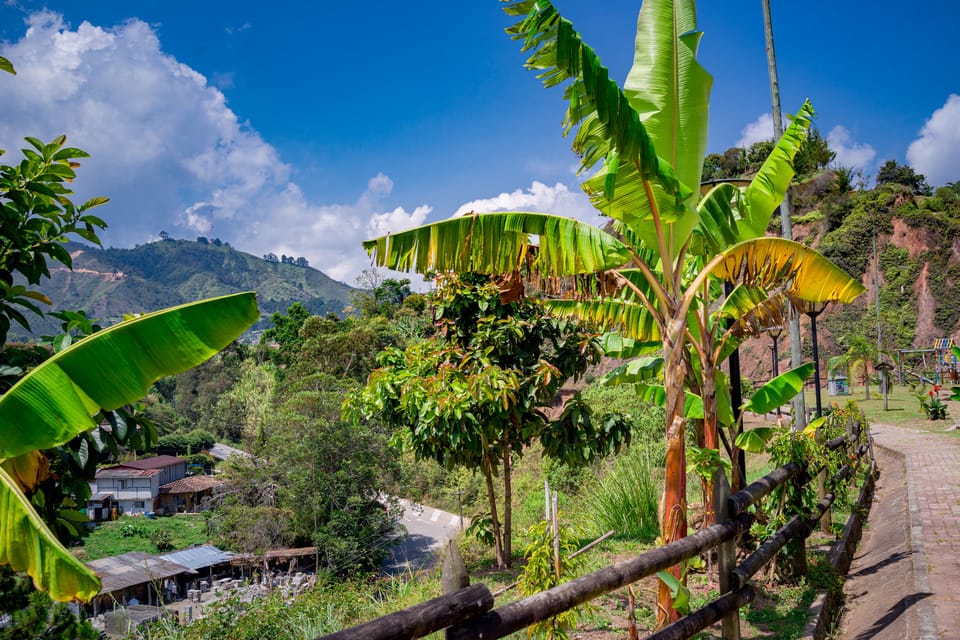This photo captures a vibrant tropical village nestled in a valley somewhere in South or Southeast Asia, taken during a sunny day with a bright blue sky adorned by billowy white clouds, particularly on the left over a tall mountain. The focal point is a small village featuring some modest tin-roofed shacks and houses with verandas. To the right, a stone brick walkway adorned with a wooden fence curves elegantly along the hillside, lined with lush palm trees. Descending from the hillside into the valley, one can see an assortment of differently built structures, alongside a road. Additionally, a partially visible colorful climbing structure suggests the presence of a playground, adding a playful touch to the serene landscape. The scene is completed by the rolling hills and the mountain range in the background, creating a picturesque tropical paradise.